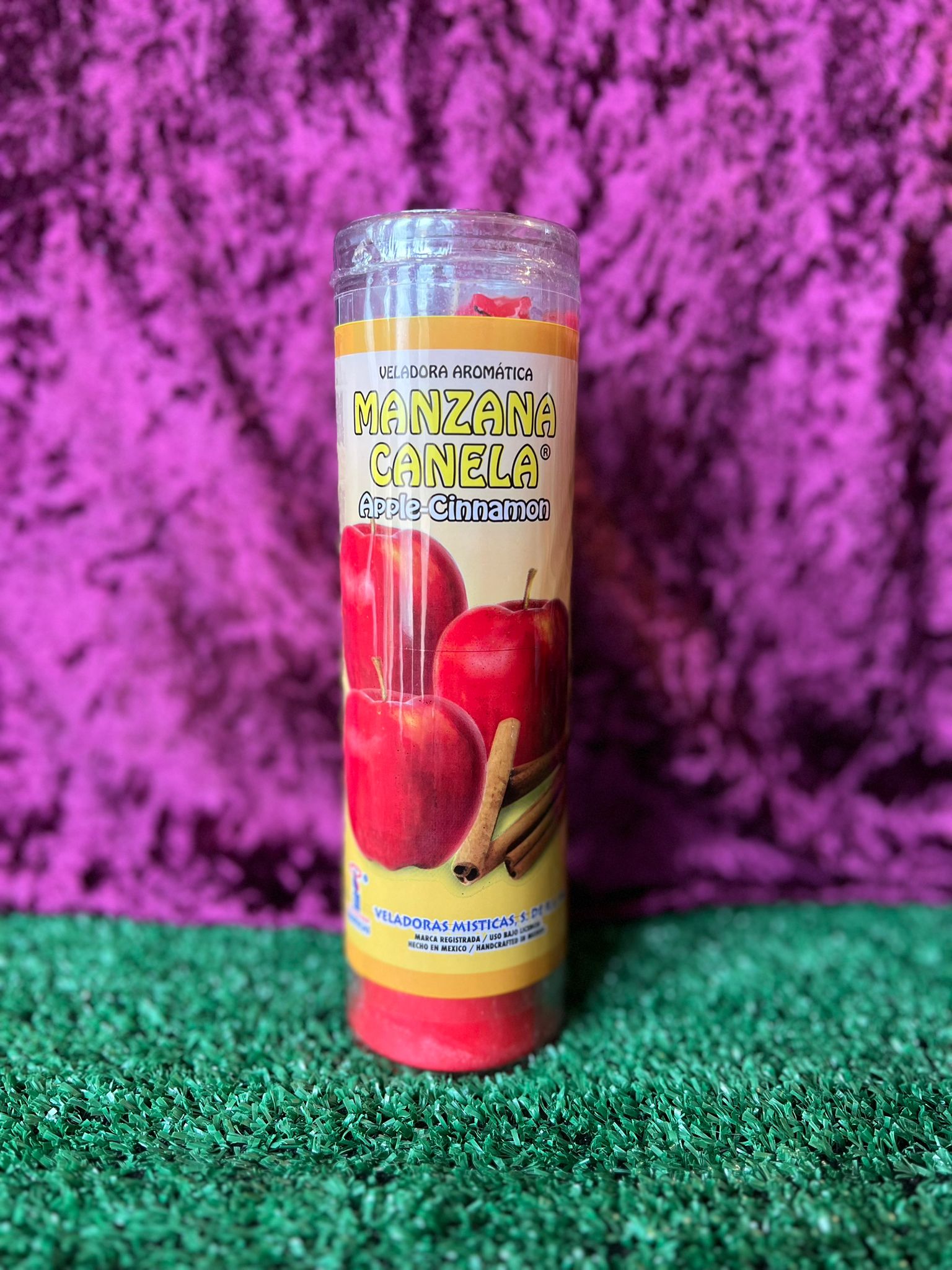The image features a tall, cylindrical candle prominently labeled in both Spanish and English. The primary text "Manzana Canela" (Apple Cinnamon) is printed in large letters, with "Apple Cinnamon" displayed beneath it in smaller white text. The label depicts three bright red apples and several cinnamon sticks resting on a yellow surface. Further details include orange stripes at the top and bottom of the label, with a gradient fading from yellow to white behind the image of the apples and cinnamon.

The candle appears to be placed upright on a green astroturf base, creating an impression of a green carpet. In the background, there is a dark purple drape or throw. The bottom of the label indicates that the product is "Made in Mexico." The top of the candle, where the wick would be visible, is out of the frame, so it's unclear whether it has been burned. The overall scene captures the essence of a meticulously arranged, yet simple still life focused on showcasing the candle's appealing apple cinnamon scent.